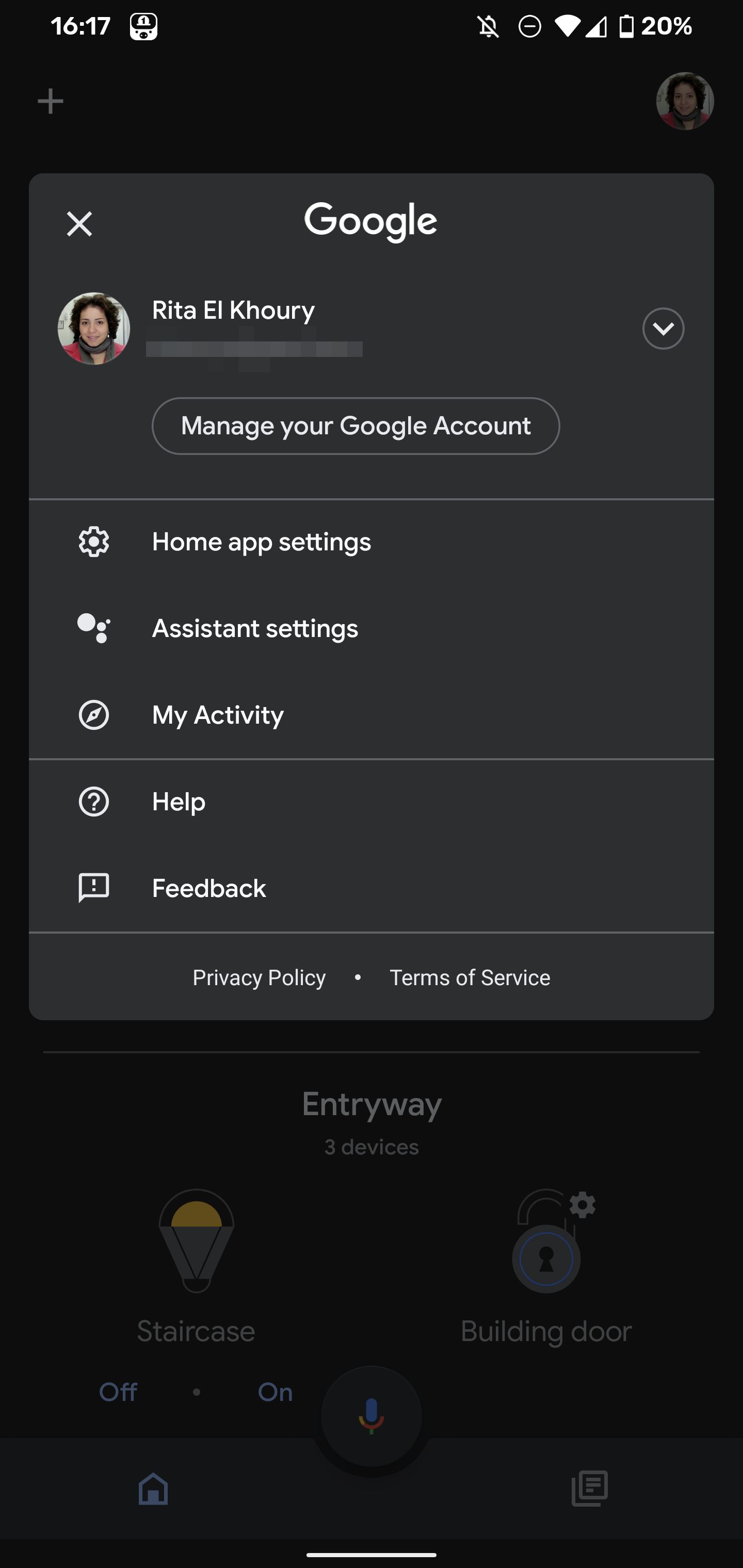The image is a screenshot from a mobile device, displaying a Google account management interface against a solid black background. In the top right corner, the military time is shown alongside a small icon. Moving left, there are standard icons for alerts (currently turned off), signal strength, Wi-Fi strength, and a battery indicator showing 20% charge.

Below this, a dark, slightly off-shade banner reads "Google" in the center with an 'X' on the left side. To the right, there's a circular icon depicting a woman identified as "Rita L. Curry," with a small drop-down arrow beside her name. 

Centered beneath it, there is a button labeled "Manage your Google account." Further down, the interface lists five rows of options for navigation, each accompanied by an icon: Home App Settings, Assistant Settings, My Activity, Help, and Feedback.

At the bottom, privacy policy and terms of service are centered with a dot between them, suggesting clickable links. The last section is grayed out, making the text barely visible, but it seems to include the word "entryway" centered, and possibly some buttons like 'Off' and 'Home' in the lower left. The visibility of these elements is significantly reduced.